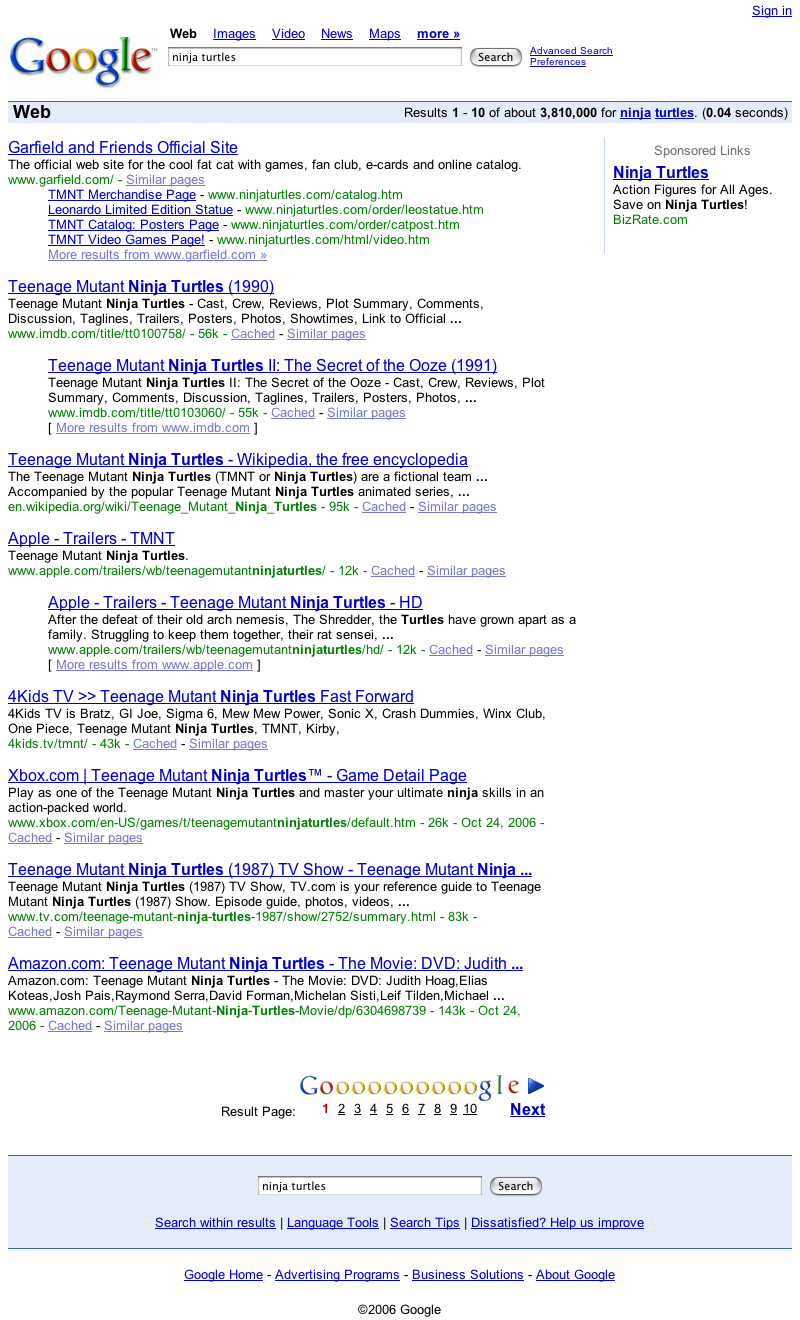In the image, a Google search results page is displayed, with the query "Ninja Turtles" entered in the search bar. The search returned approximately 3,810,000 results in 0.04 seconds. The first result oddly links to the "Garfield and Friends official site." Following that, the results pertain mostly to the Teenage Mutant Ninja Turtles franchise, starting with the 1990 movie "Teenage Mutant Ninja Turtles." The next result is for the 1991 sequel, "Teenage Mutant Ninja Turtles II: The Secret of the Ooze." Further down, there is a link to the Teenage Mutant Ninja Turtles Wikipedia page.

Subsequent results include a trailer on Apple Trailers labeled "TMT," another Apple Trailers link with an "NHD" specification, and a "4KidsTV" page featuring "Teenage Mutant Ninja Turtles: Fast Forward." There's also a link to an Xbox.com page detailing a TMNT game. The last two results feature the 1987 "Teenage Mutant Ninja Turtles" TV show and an Amazon.com listing for the TMNT movie on DVD. Each result is accompanied by a brief description and clickable links for further navigation.